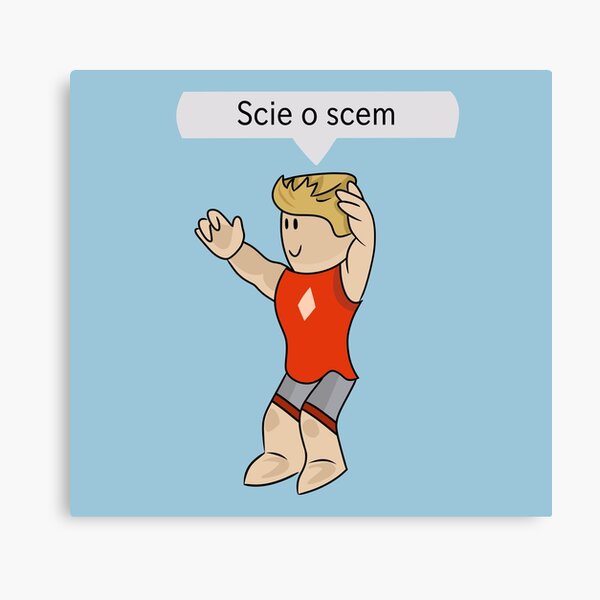The image features a character reminiscent of a Roblox or Lego figure set against an off-white background, with the main image framed by a light blue square that has shading on the left side to create a sense of depth. The cartoon character has blonde hair and simplistic black eyes, along with a smiling, nose-less face. Dressed in a white shirt adorned with an off-white diamond in the center, the character also wears gray shorts with red trim along the edges. Bending slightly with both arms raised, the character appears to be in a dynamic pose, possibly about to jump. Hovering above the character's head is a rectangular text bubble with a triangle pointer, containing the enigmatic phrase "Psy, S-C-I-E, O-Screm," giving the impression that the character is speaking or shouting these words.